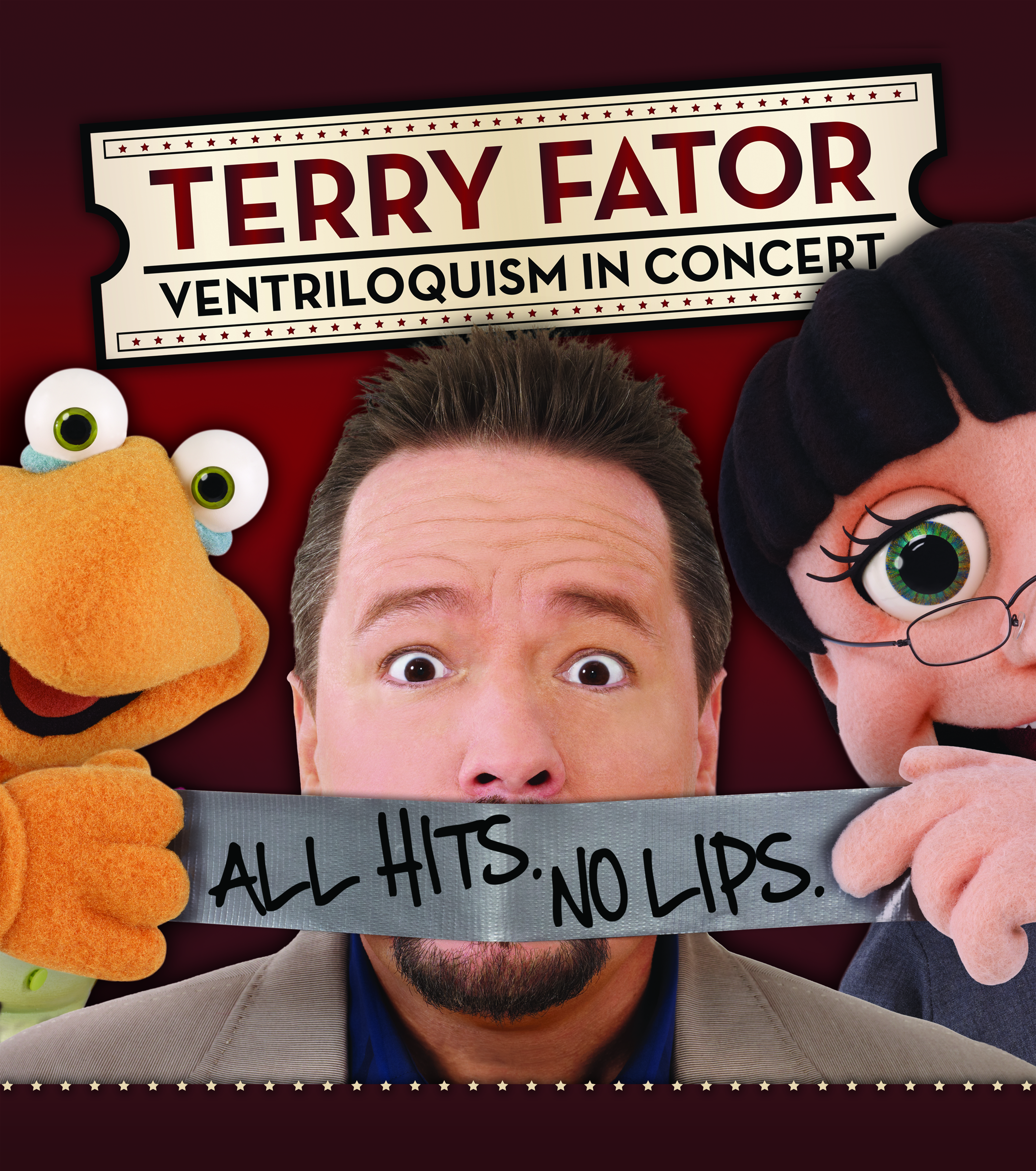The image is a detailed promotional poster featuring Terry Fator, against a red background resembling stage curtains. At the top, a ticket-shaped logo with star patterns reads "Terry Fator Ventriloquism in Concert." Below the logo, Terry Fator, a white male with spiked brown hair, is pictured wearing a light brown jacket over a blue undershirt. His expression is one of surprise as two puppets to his left and right pull a piece of silvery-gray duct tape reading "All Hits No Lips" across his mouth. The puppet on the right is a female doll with brown hair, glasses, a big green eye, and a smiling face pulling the tape with a felt hand. The puppet on the left resembles a yellow creature with large, alien-like eyes and a smiling expression, also pulling the tape. The image is framed with a dark border featuring a star pattern at the top.